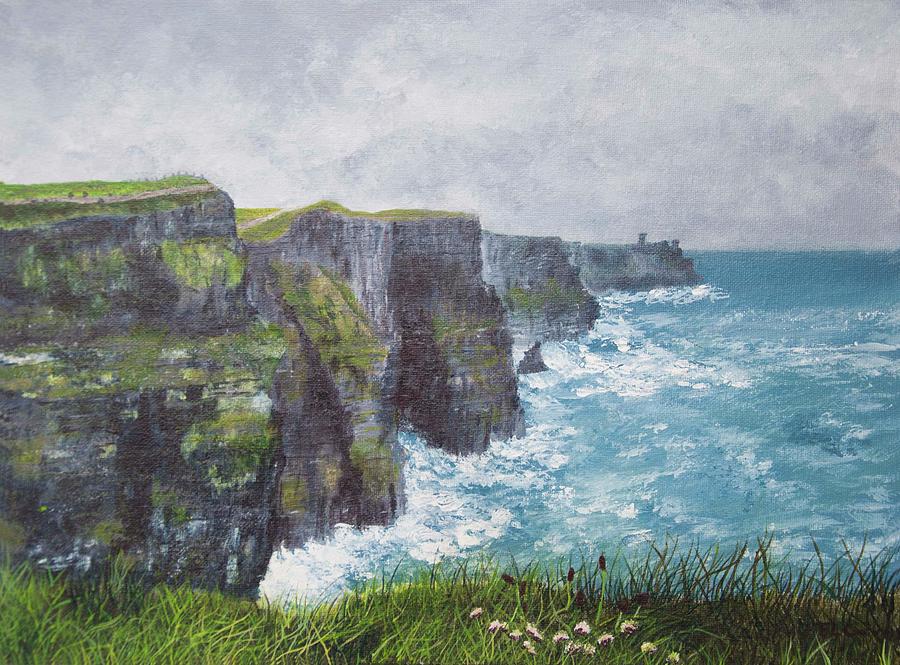The image is a pastel oil painting depicting a rugged coastal landscape. In the foreground, you stand on a grassy cliff adorned with a few white flowers, curving around from the bottom left to right. Overlooking an aqua blue ocean with choppy waves crashing and sending white caps against the rocky base of the towering dark gray and black cliffs. These cliffs, covered sporadically with grass and moss, extend outward like a peninsula into the water. In the distance, the cliffs tower above the ocean, creating a dramatic coastline. The sky above is a mottled blend of light and dark gray, adding to the painting's overall muted yet slightly vibrant color palette. The setting evokes a sense of natural beauty and timelessness, reminiscent of older oil paintings from the 60s or 70s.